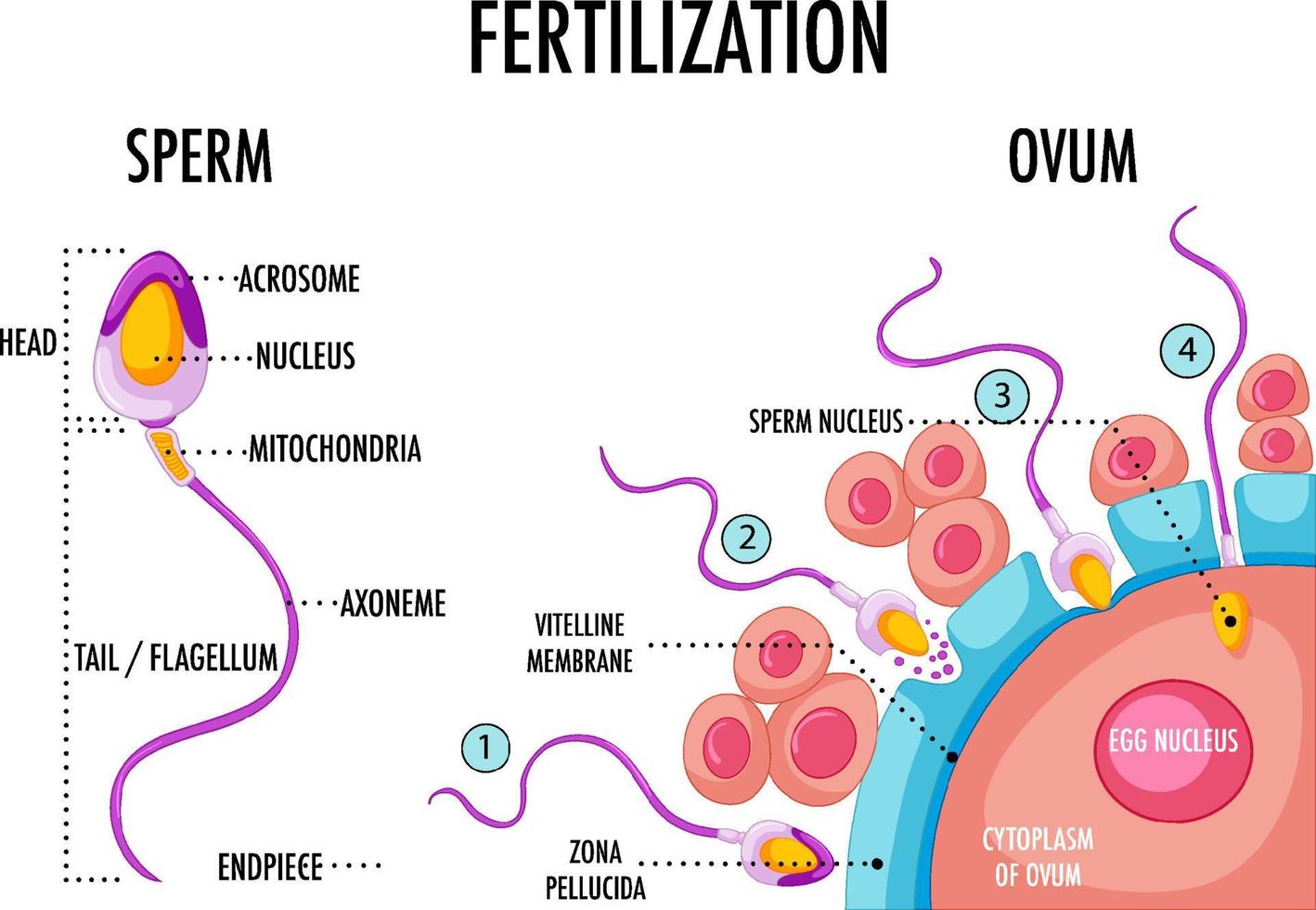This detailed diagram is titled "Fertilization" and is set against a white background, featuring two primary graphics: one of a sperm and the other of an ovum. On the left side, the sperm is illustrated in shades of purple, yellow, and orange, with labeled sections including the Head (sub-divided into the Acrosome and Nucleus), Mitochondria, Axoneme, Tail (Flagellum), and the End Piece. The right side depicts the ovum with a color scheme of blue, orange, and red. The ovum's structure is labeled with the Egg Nucleus at its pinkish-red center, surrounded by the Cytoplasm of the Ovum, the blue Zona Pellucida, and the Vitelline Membrane. The diagram visually narrates the stages of fertilization with a series of numbered steps (1-4), showing the sperm's journey: approaching the ovum, penetrating the Zona Pellucida, entering the cytoplasm, and finally the sperm nucleus heading toward the egg nucleus. Orange and red cells surround the ovum, emphasizing the detailed labeling and color-coding of the fertilization process.